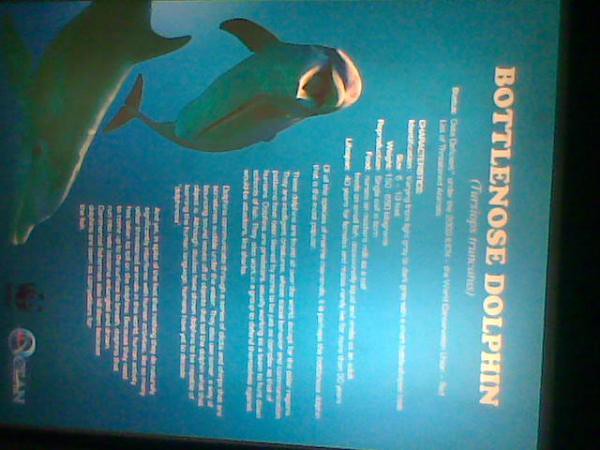The image is an advertisement for a dolphin exhibit featuring an infographic about bottlenose dolphins. The background is ocean blue, and the infographic itself is oriented sideways. Along the right-hand side, there is a black strip. The top section prominently displays the title "Bottlenose Dolphin" in white text. Below the header are images of two bottlenose dolphins: one dolphin is smiling with its mouth open, and the other dolphin is positioned off to the side. Both dolphins are grey against the blue background. The lower portion of the infographic contains extensive white text, providing detailed information about bottlenose dolphins, though the font is too small and blurry to read. At the very bottom, there is a logo with the word "ocean." The visual elements include the blue water background, white text, and the grey dolphins, highlighting the educational purpose of the sign.